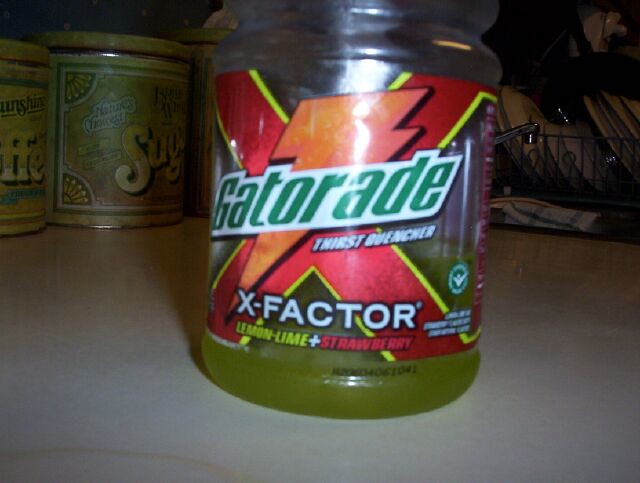In this detailed image, we observe a close-up of a partially consumed bottle of Gatorade, with approximately one-fifth of the lemon-lime plus strawberry flavored beverage remaining. The plastic container prominently features a large "X" on its label, beneath which "Gatorade" is displayed in bold green letters. Directly below, the text "Thirst Quencher" appears, followed by the designation "X-Factor" in white lettering at the bottom. The flavor descriptions, "lemon-lime" in yellow and "strawberry" in red, are clearly marked at the base of the label. In the background, slightly to the left, there is a container partially visible with the letters "S-U-G," likely indicating it holds sugar. Adjacent to this is another container showing "F-F-E," probably containing coffee. These items are all situated on a clean, white, smooth table, creating a neat and organized scene.